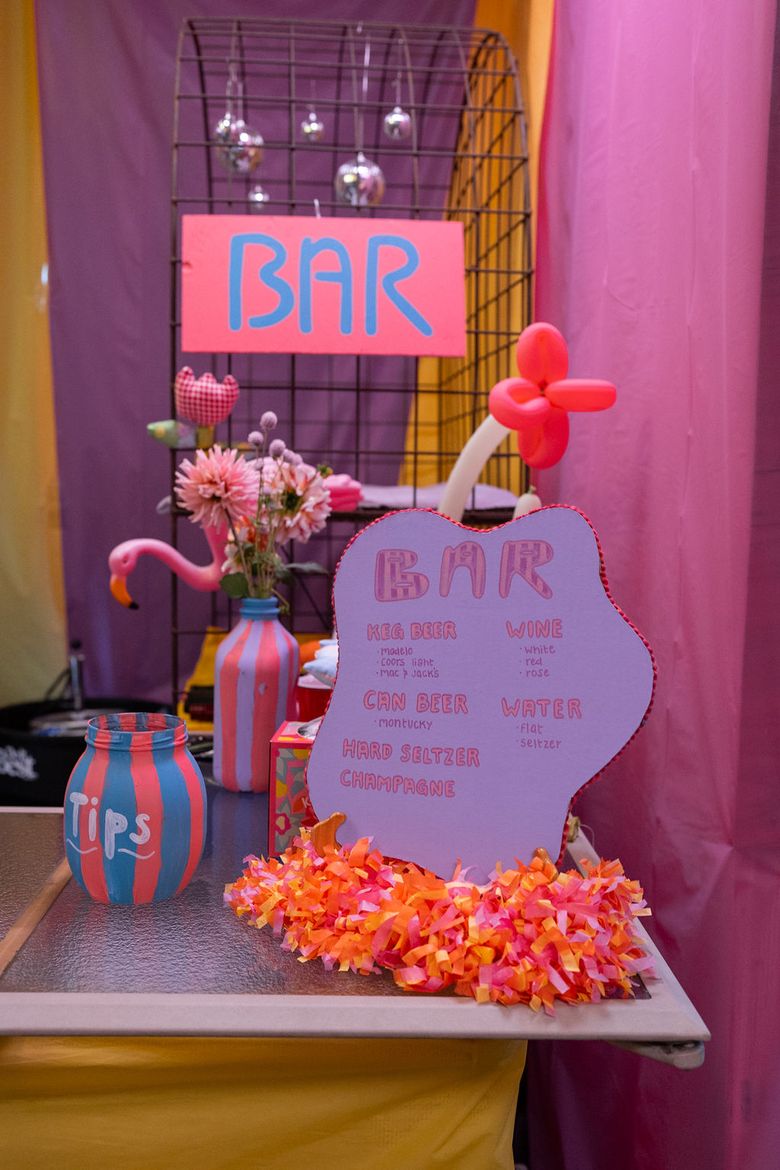In the photograph, a cozy, festive bar setup is depicted. Dominating the backdrop is a mix of purple and pink walls with yellow accents. Central to the scene is a clear glass table, accented by a yellow skirt underneath. Atop this table, there's an eye-catching lathe in orange and pink, adorned with a cutout sign that reads "Bar". This sign lists various drink options: keg beer, canned beer, hard seltzer, champagne, wine, and water. To the side, an ornate orange and turquoise jar labeled "tips" sits, with another flower-filled jar visible in the background. A whimsical pink flamingo hangs from a black wire structure overhead, contributing to the playful decor. Additionally, a sign with blue lettering on a pink background reading "Bar" is prominently displayed, complementing the overall cheerful and vibrant atmosphere.